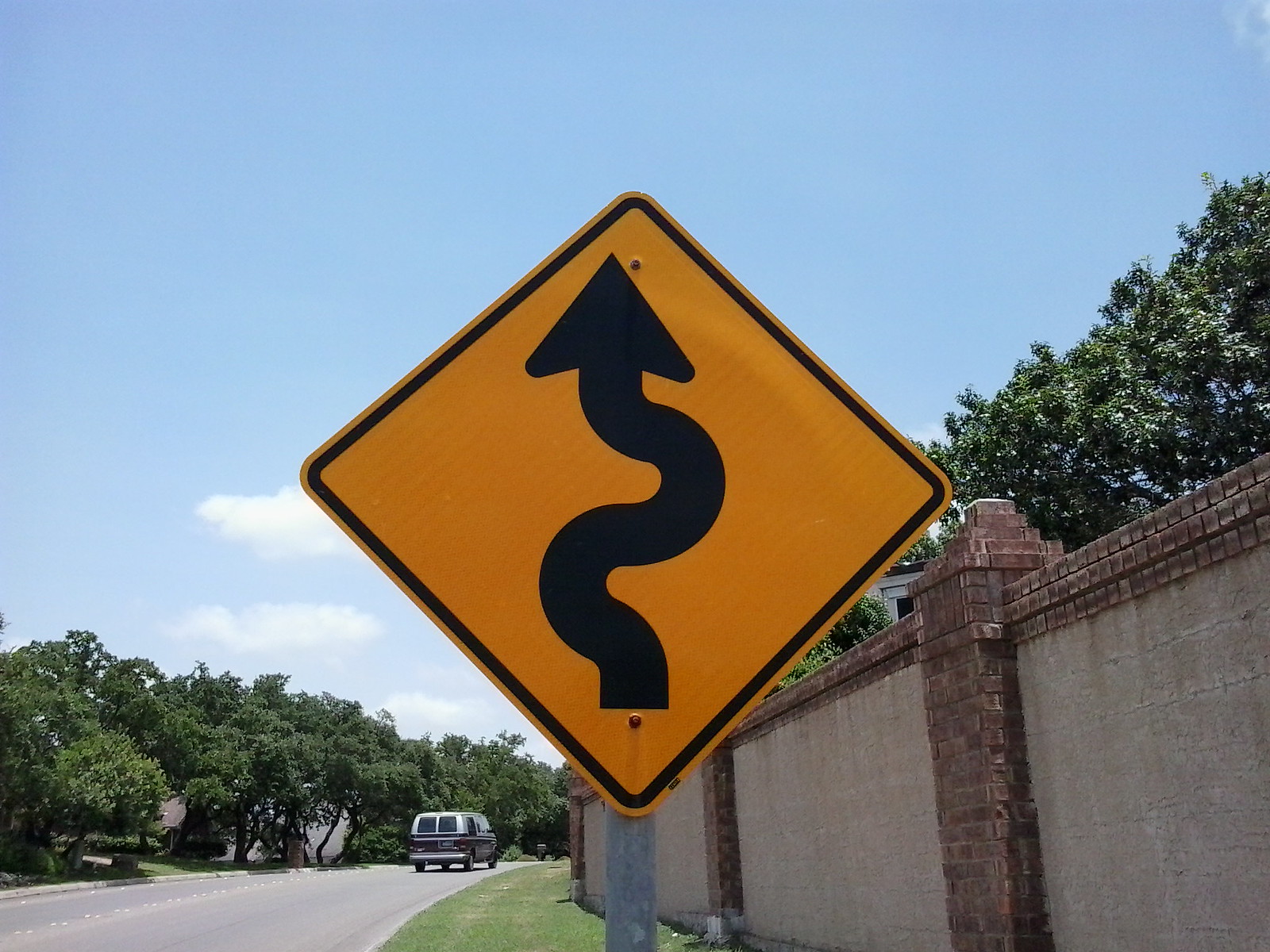"Daytime photograph showcasing a vibrant scene under a crisp, clear blue sky with fluffy white clouds. The foreground features a prominent silver metal post adorned with a black and gold sign, including intricate black trim and a curvy black arrow. A red brick and tan colored retaining wall forms a backdrop, partially obscured by lush, green trees. In front of the wall is a patch of light green grass, extending towards a light gray street. A dark van with black wheels is parked along the street, with its lower half darker and the top lighter. One of the trees in the background has a distinctive curved trunk, and behind it, the outline of a house is visible, adding to the charming suburban setting."